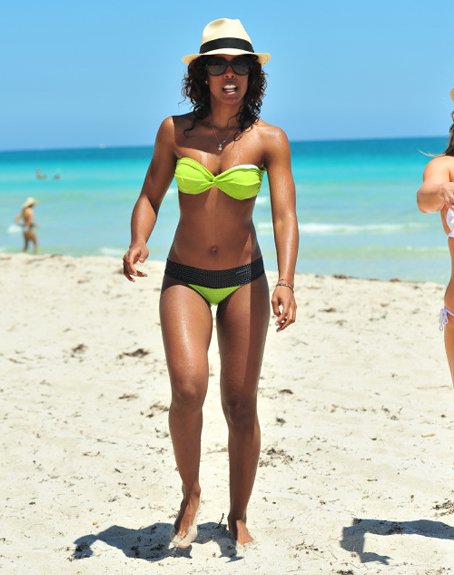The image captures a striking scene at the beach on a bright, sunshiny day. Central to the picture is an attractive African American woman wearing a neon green bikini with a black band around the bottom. She has a medium skin tone and wavy dark hair, accessorized with a cream-colored hat featuring a black band and stylish sunglasses. She is standing upright and appears to be walking barefoot, her left foot slightly off the ground, revealing the sand on her feet. She also sports a necklace and a bracelet on her left arm. Her mouth is open, perhaps mid-conversation or in a candid moment of joy. In the background, there are people and a picturesque view of the beach, with clear blue skies and a beautiful ocean. To the right, partially cut off from the picture, there's another woman in a white bikini, standing with her long hair and right arm extended. Further in the background, to the left, a person is seen wearing a cowboy hat. The image exudes a lively, carefree beach atmosphere.